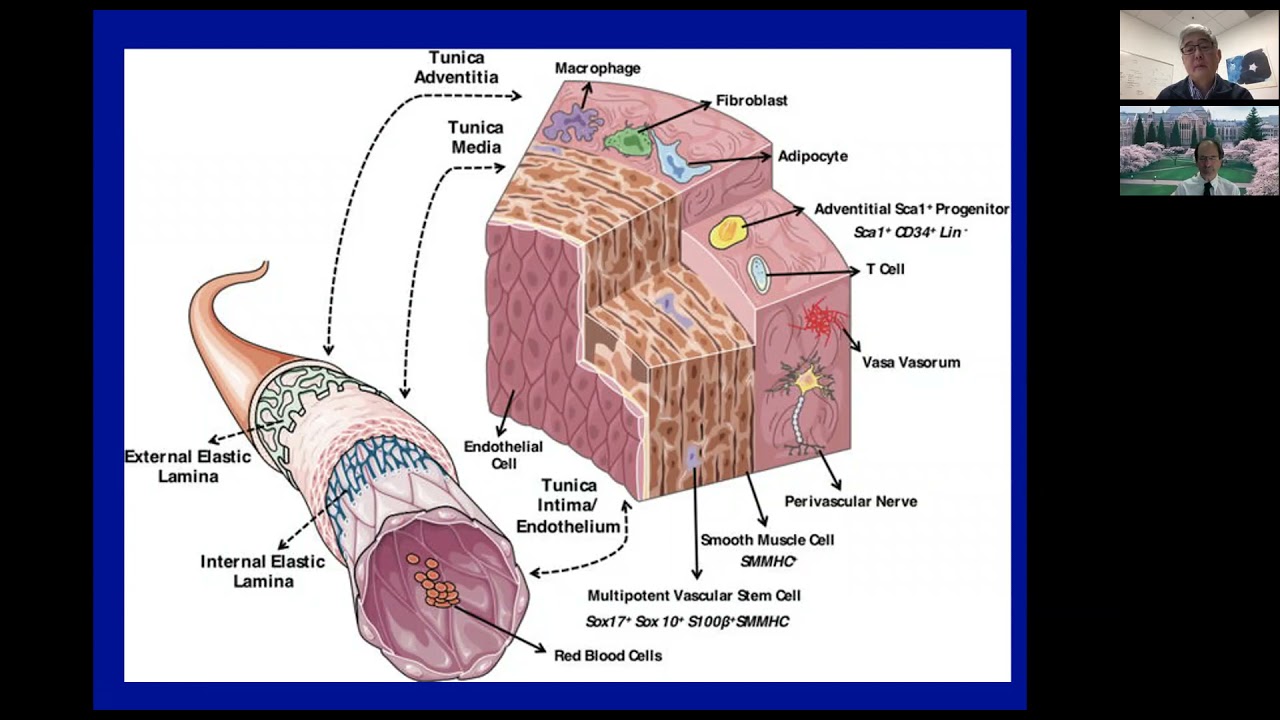This scientific illustration features a detailed cross-section of a vascular structure on a white background. The image is subdivided into multiple layers, each meticulously labeled with terms like fibroblast, adventitial progenitor, vasa vasorum, endothelial cell, internal elastic lamina, external elastic lamina, tunica adventitia, tunica media, perivascular nerve, smooth muscle cell, red blood cells, adipocyte, and macrophage. The diagram elaborates on the complex architecture of blood vessels, showing how each layer and cell type contributes to the overall structure. The lower part of the image displays a longitudinal view, revealing a tube-like structure with layers peeled away to expose the inner components, such as the red blood cells traveling through the lumen. In the top right corner, there is an inset featuring a cross-sectional view of the tube, providing a different perspective on the anatomical details. Additionally, the outer border of the image is gray-black with a blue inner frame. In the top right corner, two small screens depict individuals engaged in an online meeting, suggesting a collaborative scientific discussion.